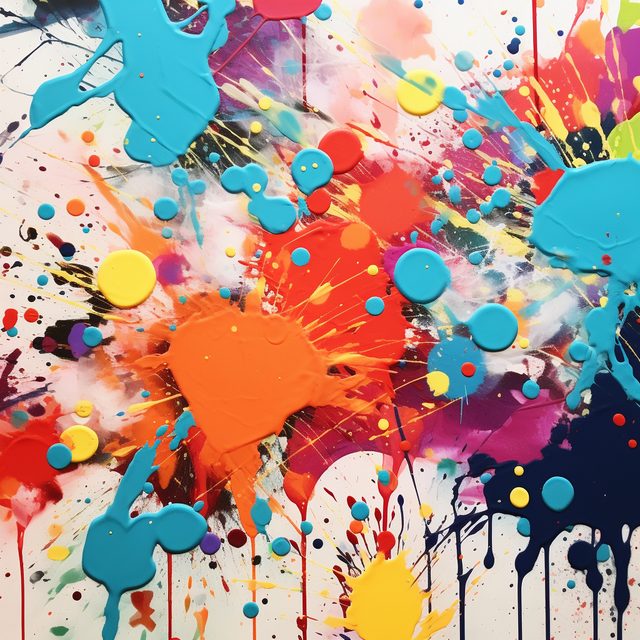The image is a captivating and artistic photograph showcasing a vibrant array of paint splatters on an off-white surface. The surface is adorned with an eclectic mix of colors, including shades of yellow, navy, red, orange, teal, magenta, purple, light pink, white, gold, black, plum, green, and a striking white-orange hue. The paint splatters vary in shape and size, ranging from circular and oval puddles to spontaneous, scattered droplets. Some sections exhibit a watercolor-like effect, where the pigments blend and merge fluidly. The overall impression is one of unrestrained creativity, as if the artist playfully flung their paintbrush to allow the colors to land where they may. The aesthetic is further enhanced by certain areas where the paint appears to have a melted or marbled texture, adding depth and intrigue to the composition. The seemingly chaotic splashes of color coalesce into a mesmerizing and dynamic visual experience, making it a feast for the eyes.